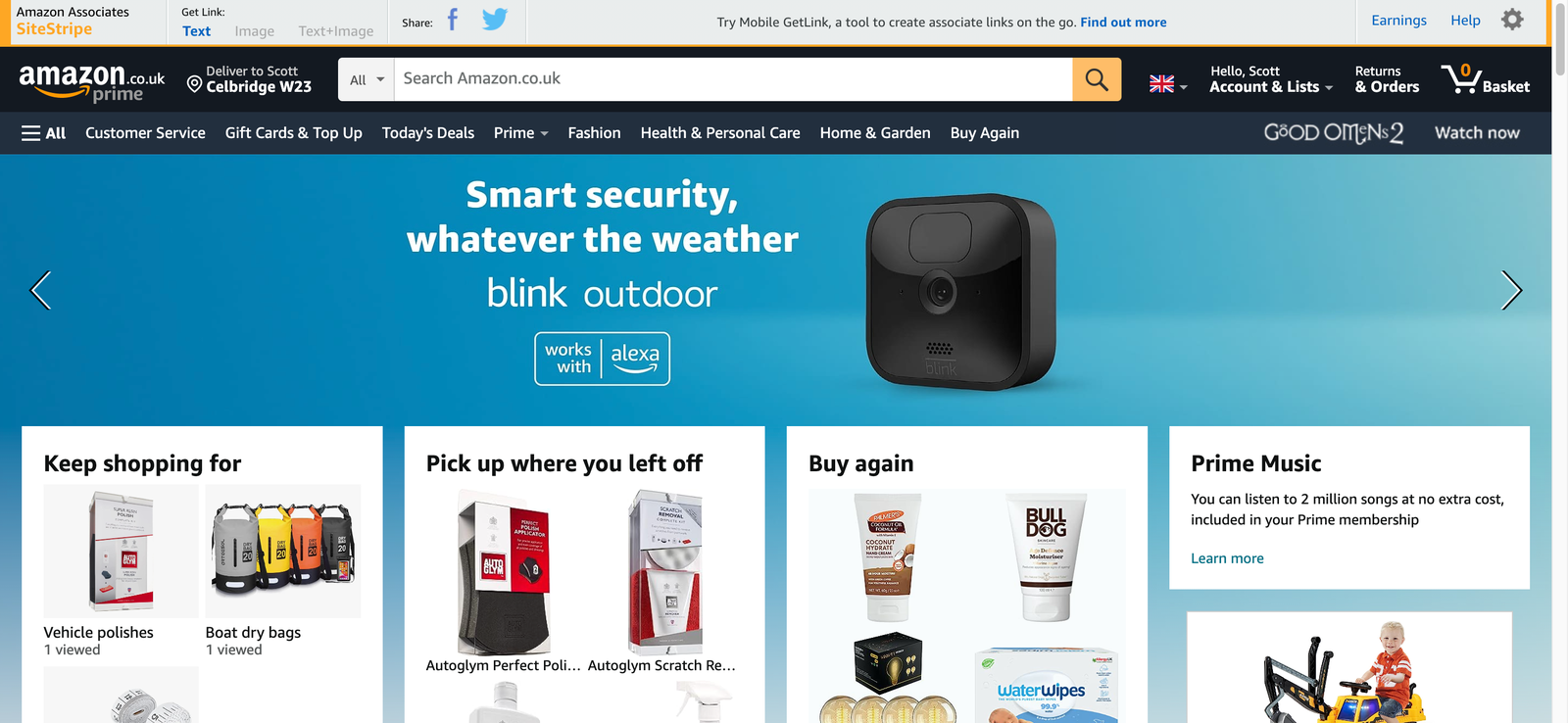**Detailed Caption:**

The image is a detailed screenshot of a web page, likely from an Amazon Associates account. At the very top of the screen, there's a gray navigation bar. In the top left corner, the text "Amazon Associates" is displayed, with "SiteStripe" written in orange beneath it. To the right, there is a "Get Link" option with various choices: text, image, text + image, and sharing options for Facebook and Twitter. Further to the right, there is an option for "Try Mobile Get Link," a tool designed to create associate links on the go, accompanied by a "Find out more" link.

On the far right of the gray bar, there are icons and options for "Earnings," "Help," and a gear icon for "Settings." Below this top bar and aligned to the left, various elements of the Amazon.co.uk interface are visible, including the text "Amazon.co.uk," "Prime," "Deliver to Scott," and "Sellbridge, W23." There's a search bar that reads "Search Amazon.co.uk," followed by "Hello, Scott," "Account and Lists," "Returns and Orders," and "0 Basket."

The menu options listed include "All," "Customer Service," "Gift Cards & Top Up," "Today's Deals," "Prime," "Fashion," "Health & Personal Care," "Home & Garden," and "Buy Again."

Below the gray bar, the background transitions to blue, featuring an advertisement for a black, square-shaped device, which appears to be a camera with a button on top. The white text to the left of the device reads: "Smart Security, Whatever the Weather, Blink Outdoor," and notes compatibility with Alexa.

At the bottom of the image, there are additional ads showcasing various products, including bags and creams.